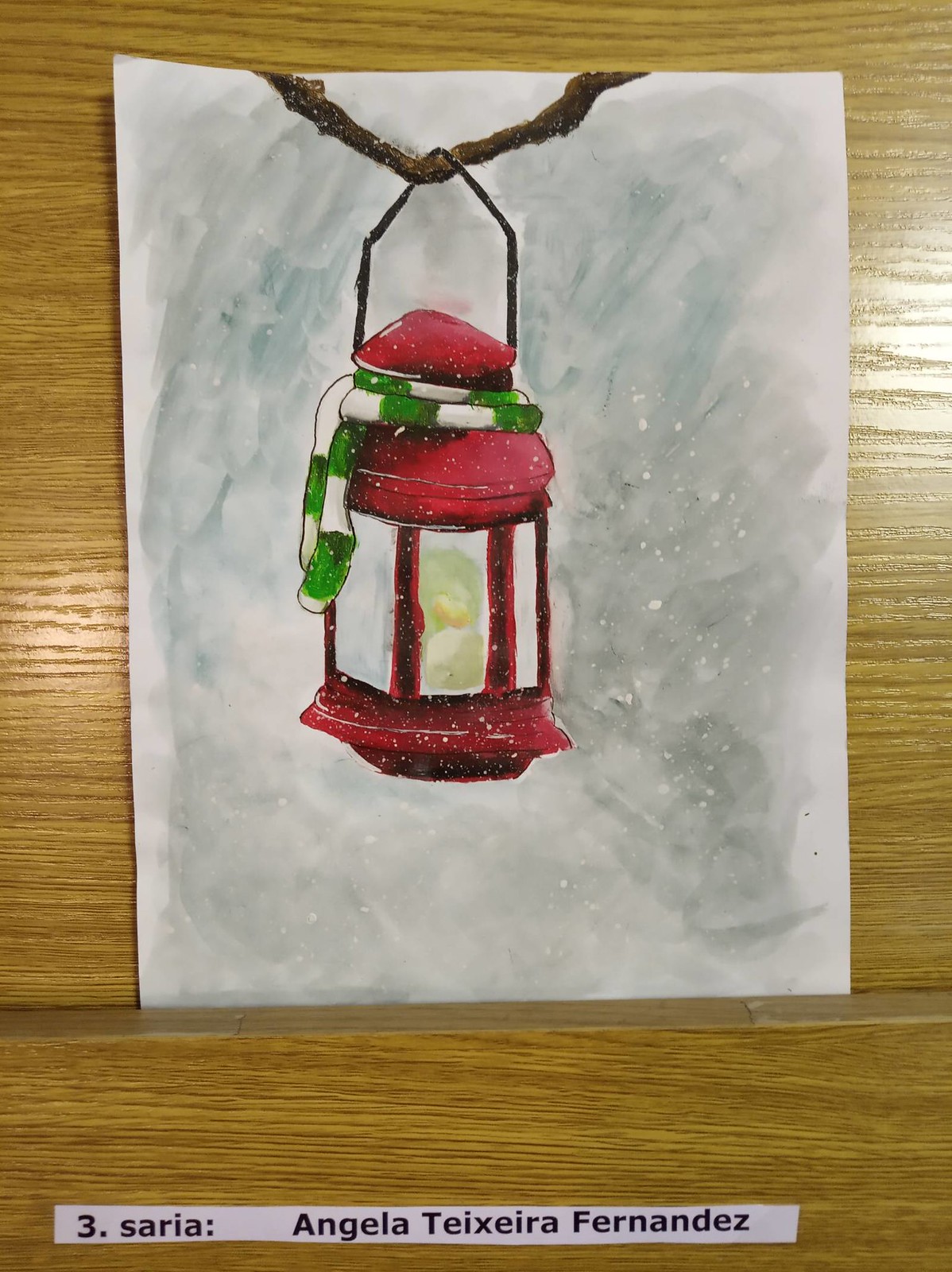This image captures a meticulously crafted artwork, likely a watercolor painting or colored drawing, displayed on a light brown wooden surface. The white sheet of paper showcases a red lantern, intricately hanging from a dark brown branch via a black metal handle. This lantern, glowing warmly from the flame inside, features clear glass panels and a dome-like top draped with a green and white striped scarf. The background is a swirling mix of grays and dark blues, dotted with white circles resembling falling snow. At the bottom of the artwork, a white banner bears the inscription "3 Saria," and slightly below, the artist's name, "Angela Teixeira Fernandez," is elegantly written.